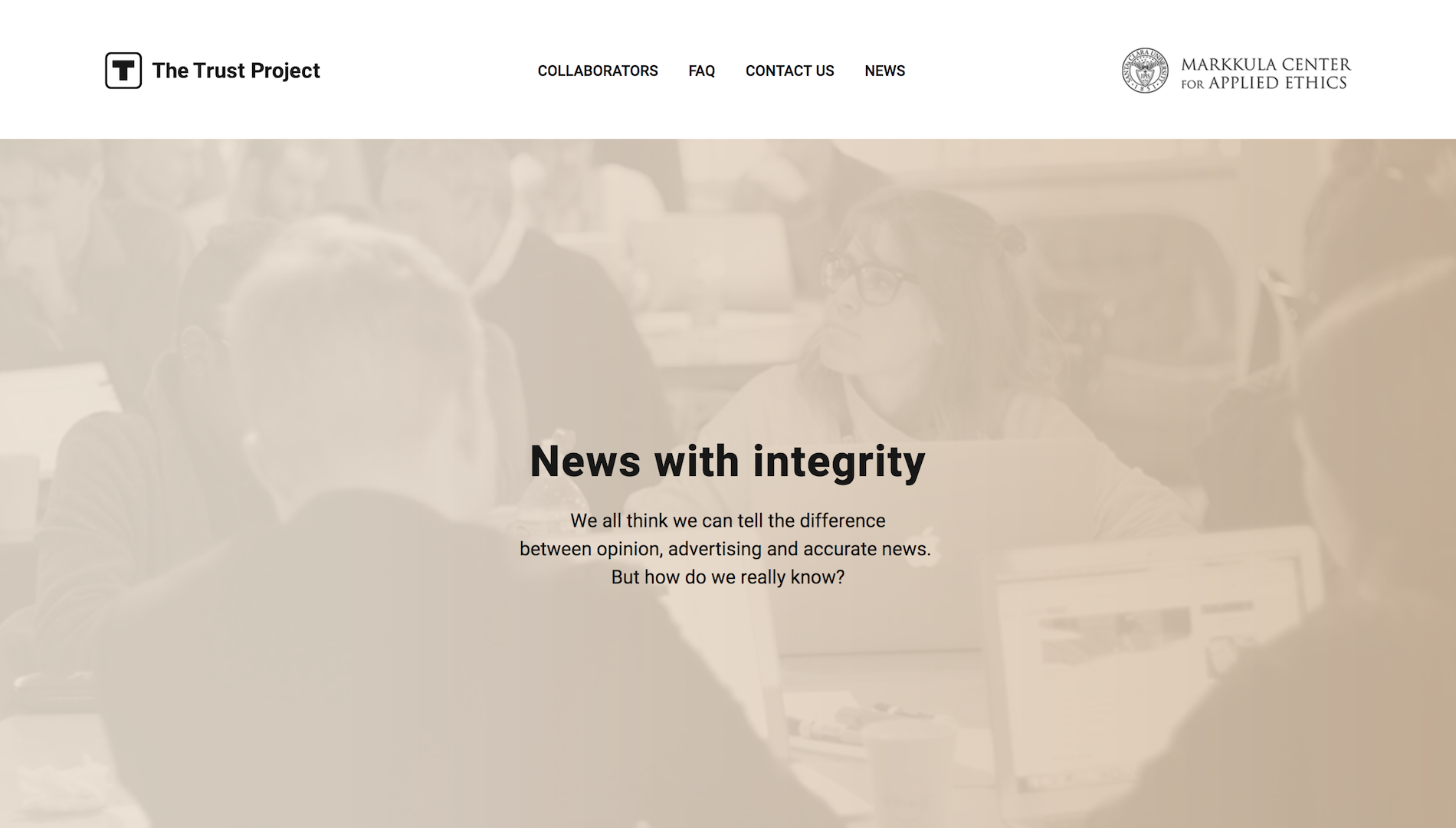A screenshot of a desktop application showcases "The Trust Project" with a distinctive black letter "T" enclosed in a square as its company logo on the top left. In the center of the screen, the navigation bar features tabs labeled "Collaborators," "FAQ," "Contact Us," and "News," all in a uniform black font. On the top right corner, it displays "Markkula Center for Applied Ethics" next to its company logo, which depicts an intricate design of a circle with an eagle clutching a crown beneath its talons.

Dominating the middle of the screen, a slightly faded background image spans from left to right, capturing a scene of a woman in glasses facing right, presumably a colleague. She is seated at a long table alongside another woman who is operating a laptop in front of her. The laptop screen is not discernible in detail. Around them, other men and women are present, though their faces are blurred, suggesting a perspective or bokeh effect, with the woman in glasses being the focal point of the sharpest clarity. 

Prominently, in larger black font in the center, the text reads, "News with Integrity." Beneath that, a smaller text prompts, "We all think we can tell the difference between opinion, advertising, and accurate news, but how do we really know?" The background image exhibits a gradient transition from a grayish-white hue on the left to a sepia-like brown on the right, enhancing the visual depth and focus.